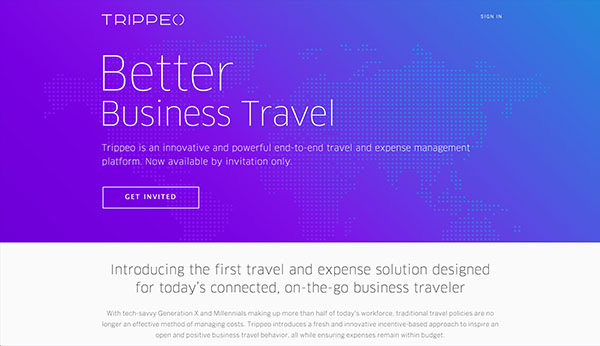The image features a background with a gradient rectangle that transitions from purple on the left to blue on the right. Behind this gradient are subtle dot patterns that are more visible on the blue side but barely noticeable on the purple side. The blended blue side even hints of purple towards the bottom. 

Prominently displayed within this gradient rectangle is the text "TRIPPEO". To the right of this headline are some smaller, unreadable words. Below the main title, there's a tagline that reads, "Better Business Travel." 

Underneath this tagline, it further explains: "GPO is an innovative and powerful end-to-end travel and expense management platform, now available by invitation only." This description is followed by a white outlined rectangle containing the text "Get Invited."

Beneath this call-to-action box, another sentence introduces the service: "Introducing the First Travel and Expense Solution Designed for Today's Connected On-The-Go Business Traveler."

The very bottom of the image contains approximately three lines of smaller text, which is too small to decipher. All these elements are designed to convey a cohesive and professional message about a cutting-edge travel and expense management platform targeted at modern business professionals.